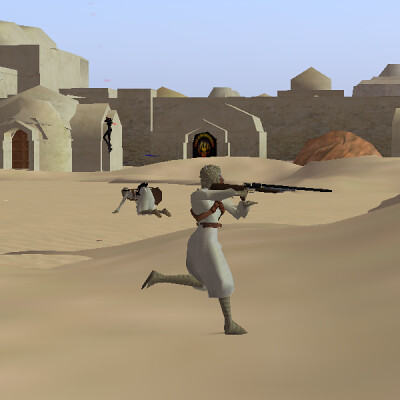In this image, which appears to be a screenshot from a late 90s or early 2000s video game, a character is depicted running with a long rifle pointed to the side. The graphical style and quality suggest the game's vintage era. The scene unfolds in a desert environment under a clear blue sky, indicating midday. In the background, there are additional structures, including a distinct black door adorned with gold trimmings. Another character is seen on their hands and knees, seemingly attempting to rise. This visual captures a moment of action and tension, characteristic of the era's game design aesthetics.